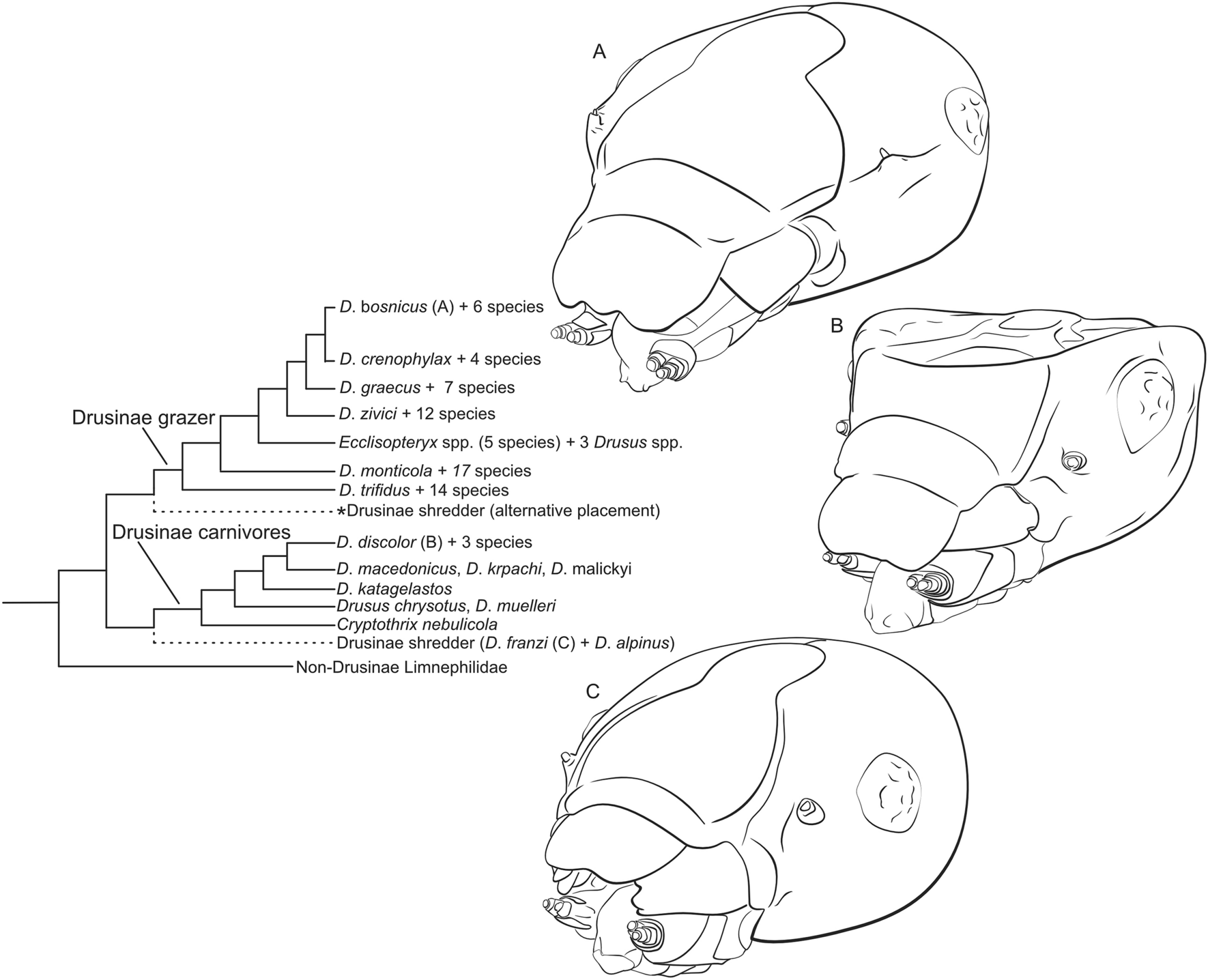This scientific illustration presents detailed cross-sectional views of skulls from various carnivorous species. The left side features a legend that categorizes each diagram, labeled A, B, and C from top to bottom. The legend provides taxonomic classifications, listing the genus and species of each depicted animal.

- **Figure A**: Features the skull of "Drizzen egg razor."
- **Figure B**: Illustrates the skull of "Drizzen egg carnivores."
- **Figure C**: Depicts another categorized carnivorous skull.

Adjacent to these sections, the diagram lists approximately 15 different genera and species, offering a representation of the diversity within these classifications. Each cross-section unveils the structural intricacies of the skulls, although the legend provides limited details on the unique characteristics of each genus and species. The descriptions and visual aids collectively enhance our understanding of these carnivorous species' skull anatomy.